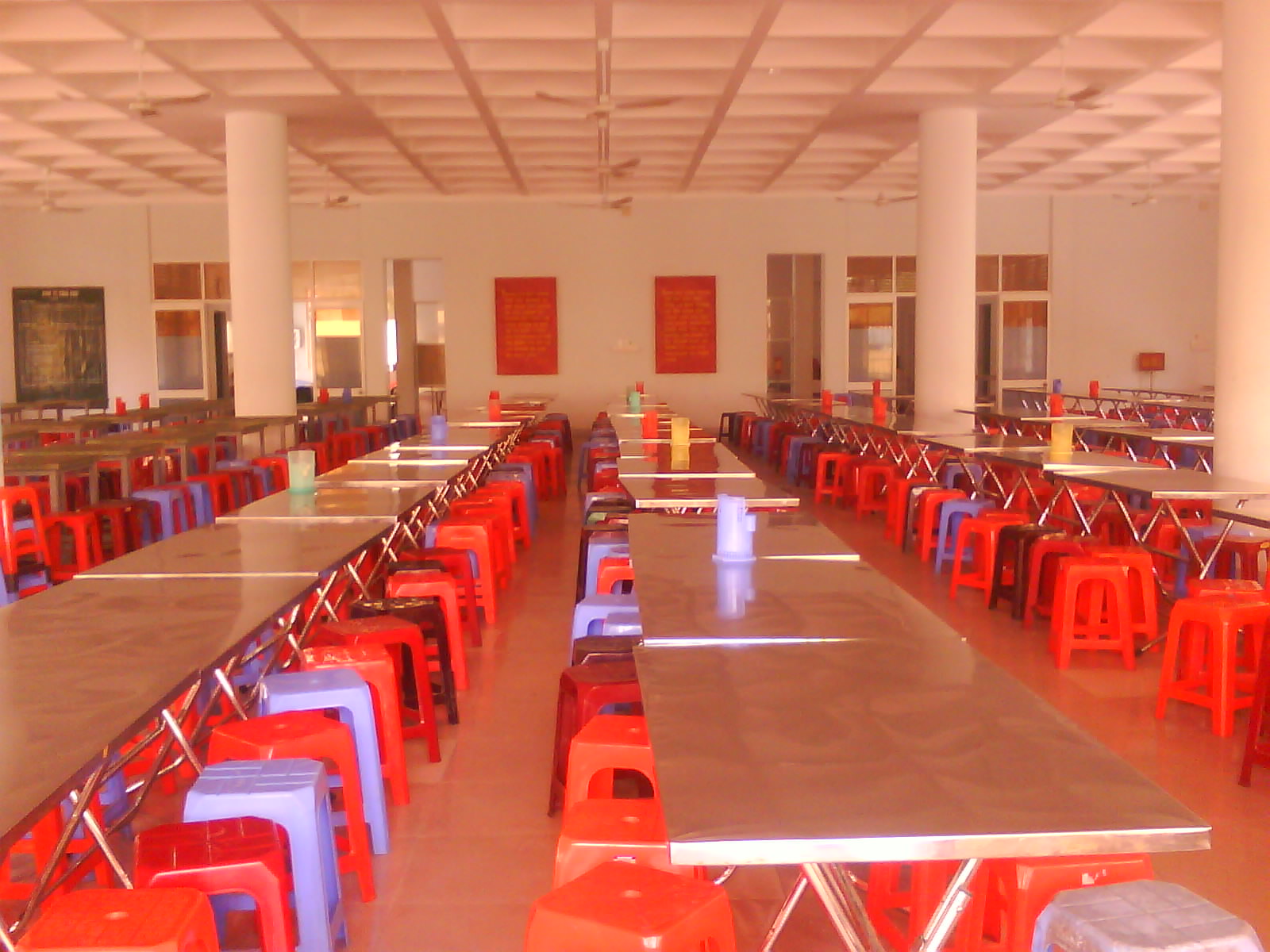The image is a colorful photograph of what appears to be a school cafeteria or preschool lunchroom, captured in landscape orientation. The room features a long array of tables arranged vertically from the bottom of the frame toward the center. These tables have a fake wood surface with silver metal edges and sturdy metal legs. Surrounding the tables are rows of plastic stools in a vibrant mix of bright orange, pale blue, and predominantly red colors, with a few brown and black stools scattered throughout. The lighting in the room accentuates the vivid hues of the stools. On some of the tables, there are objects that appear to be plastic water pitchers, although details are not clear. The ceiling is visible and the room is predominantly beige, with large columns adding to the structural design. In the background, bright orange posters adorn the walls, and red blinds cover the windows. Additionally, doorways on both the left and right sides of the room lead out to hallways, further suggesting the room's function as a communal eating area.